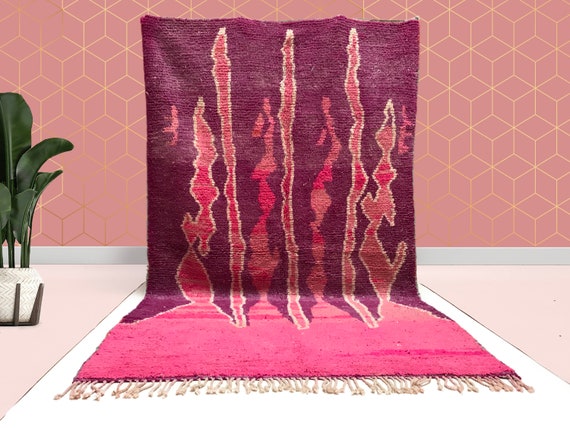The image displays a detailed and intriguing scene, with a central rug that hangs from the wall and drapes onto the floor, creating a seamless continuation from vertical to horizontal. The rug begins with a dark shade of purple at the top which gradually transitions into a lighter shade of purple and culminates in a pink hue towards the bottom. The area at the bottom features golden tassels that gently rest on the floor. This rug is notably adorned with intricate, lighter shapes that resemble thunderbolts or potential seaweed-like patterns starting from the pink section and extending upward into the purple.

The backdrop features a pale pink wall that gives a modern, digitally-rendered appearance due to its three-dimensional geometric pattern of interconnected golden cubes. The floor beneath the rug is a soft peach color, complementing the overall pastel theme of the scene. Additionally, there is a second white rug peeking out under the primary hanging rug, lying on the white carpeted floor.

To the left side of the image, a lush green plant is seen in a white vase, contributing vibrant greenery to the otherwise pastel-dominated palette. The plant has three to four large leaves adding a natural contrast to the geometric precision of the wall and the soft textures of the rugs.